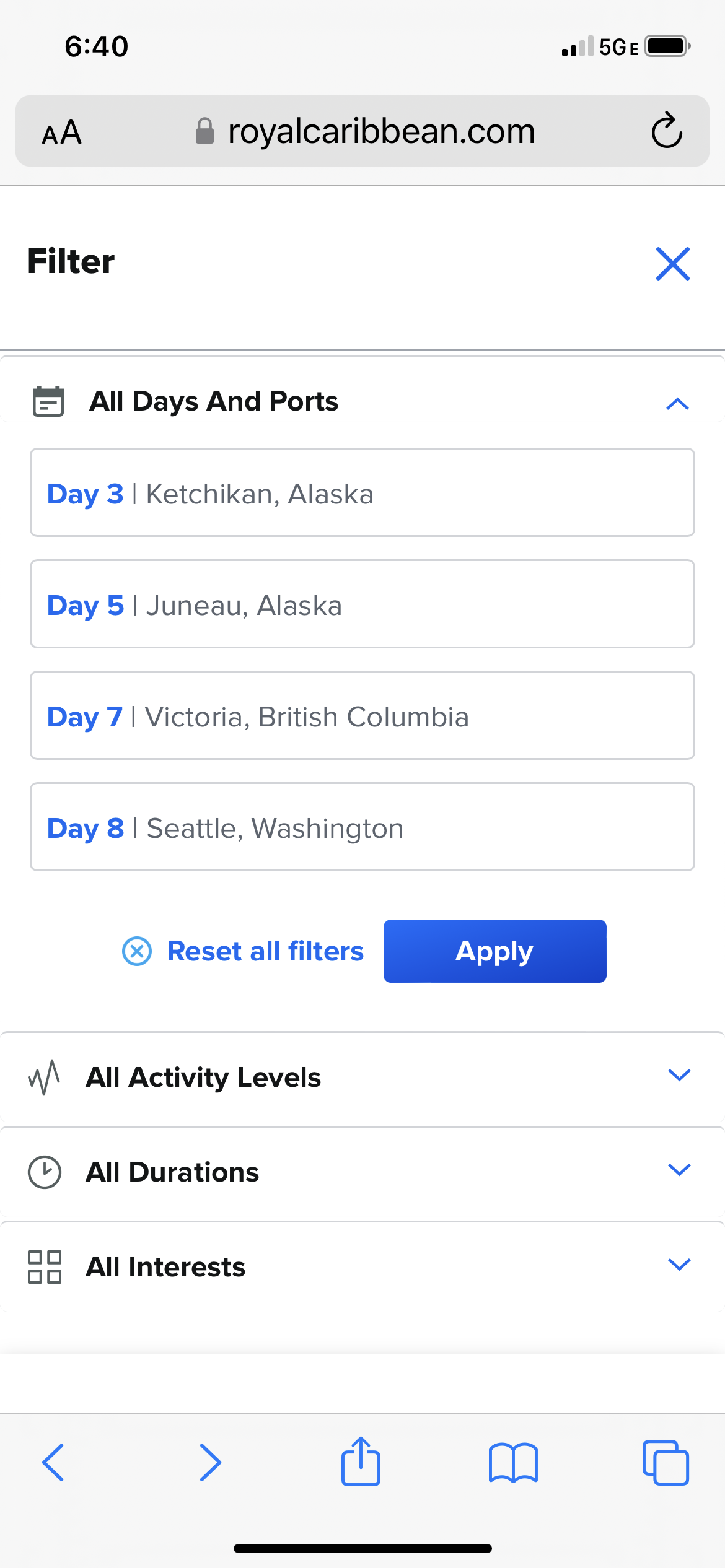A detailed screen capture of a smartphone interface. The phone displays the time as 6:40 and is connected to a 5G network with a full battery. The screen shows the website royalcaribbean.com, with filters set for "All Days and Ports." The itinerary visible includes:

- Day 3: Ketchikan, Alaska
- Day 5: Juneau, Alaska
- Day 7: Victoria, British Columbia
- Day 8: Seattle, Washington

Options to reset or apply all filters are prominently displayed. Below these, additional filter categories are available, including "All Activity Levels," "All Durations," and "All Interests." Icons at the bottom of the screen include a left arrow, a right arrow, a box with an upward arrow (likely for sharing or uploading), a stylized open book, and two overlapping boxes, indicative of a multi-window or compare feature. This screen appears to be part of the cruise booking process for a round-trip itinerary to Alaska with a return to Washington.